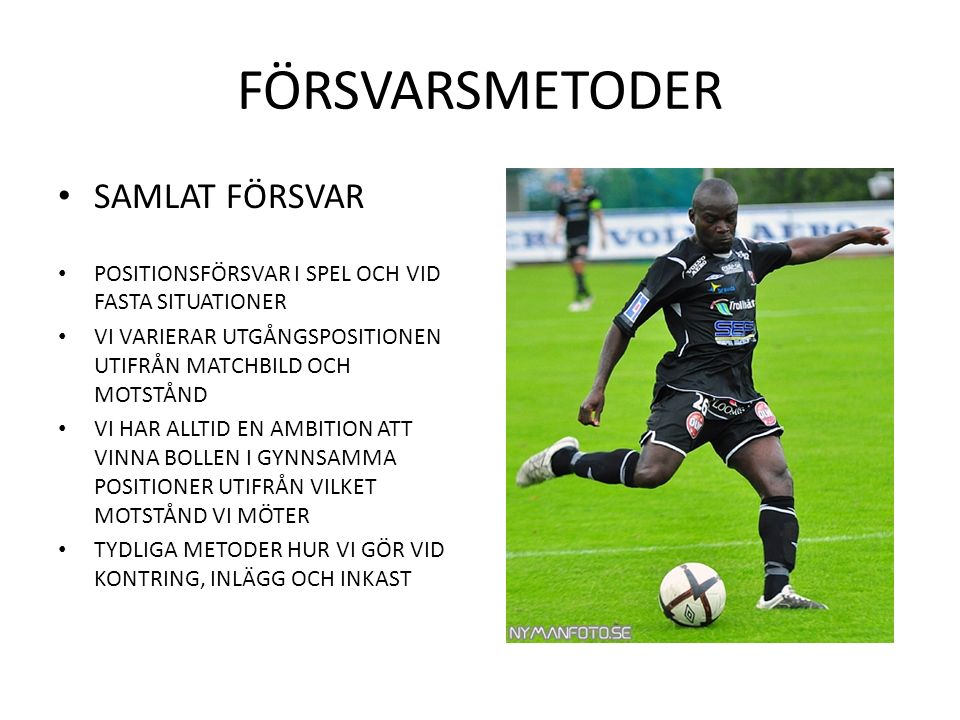In this detailed outdoor soccer field image taken during the day, a black soccer player is captured mid-action, preparing to kick a soccer ball. The player, donning a sleek black jersey adorned with sponsor logos that include "AERO" and "SES", and the number 26, stands out against the grassy pitch. His uniform is complete with black shorts, tall black socks, and white or gray sneakers. The player has minimal hair, appearing almost bald. 

In the background, the field stretches out with another player, who appears to be white and similarly attired, visible in a blurred form. An advertising wall behind them displays the partially obscured text "VOBVOEAERO" in white and blue. The lower left-hand corner of the image features the watermark "NYMANFOTOSE".

To the left side of the image, forming an infographic layout, is a series of bullet points written in a foreign language. The text includes phrases such as "FORSVARSMETODER," "SAMLATFORSVAR," and "BOLLEN," although much of the text remains unreadable or blurred. This detailed composition highlights the dynamic moment on the soccer field while providing a glimpse into the context and sponsorship surrounding the sport.